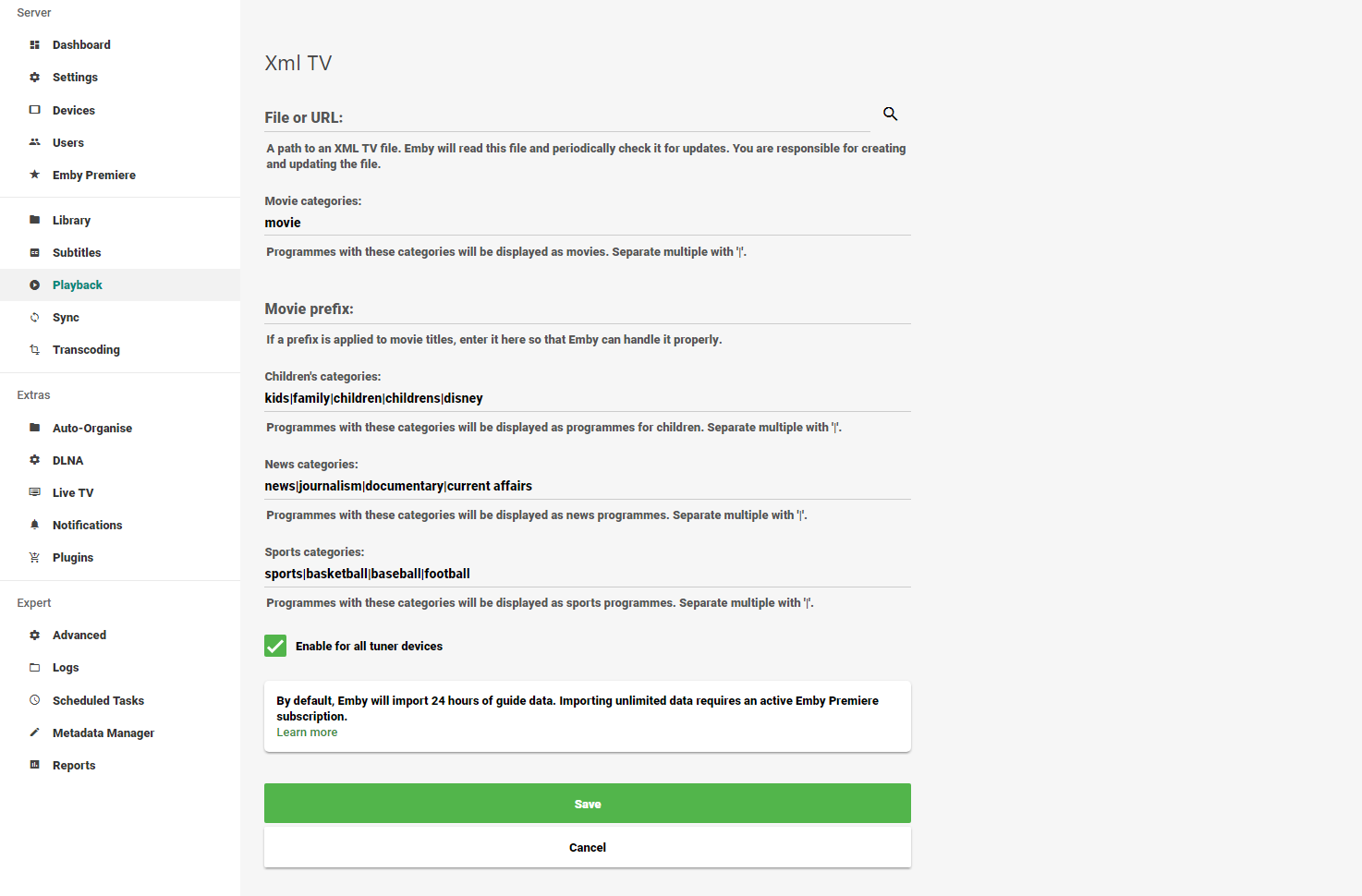This screenshot captures a settings page of a computer application with meticulous detail. The main background of the page is light gray, providing a neutral backdrop against which the white sidebar on the left stands out. At the top of the sidebar, in dark gray text, the word "Server" is prominently displayed.

Underneath "Server," a series of indented lines begin, each starting with a distinctive icon followed by black text, categorizing various sections. These sections are divided by thin, light gray separator lines for clarity.

The first section under "Server" lists:
- "Dashboard"
- A cog icon followed by "Settings"
- A rectangular icon with "Devices"
- An icon of two people for "Users"
- A star icon with the label "MB Premiere"

A separator line follows, leading into the next set of options:
- A file folder icon with "Library"
- A square with white quotation marks labeled "Subtitles"
- A donut icon with the word "Playback"
- A refresh icon for "Sync"
- An icon that is indiscernible, labeled "Transcoding"

Another separator line divides these from the subsequent section. At the top of this section is "Extras" in light gray text. The list continues with:
- A file folder icon for "Auto-organize"
- A cog icon labeled "DLNA"
- A TV icon for "Live TV"
- A bell icon for "Notifications"
- A shopping cart icon leading to "Plugins"

Yet another separator line marks the transition to the final section, labeled "Expert" in light gray text at the top left. Under "Expert," the options are:
- A cog icon with "Advanced"
- A file folder icon labeled "Logs"
- A clock icon indicating "Schedule Tasks"
- A pencil icon at a 45-degree angle for "Metadata Manager"

The layout is well-organized, with each section and item clearly delineated by icons and separator lines to enhance user navigation and clarity.